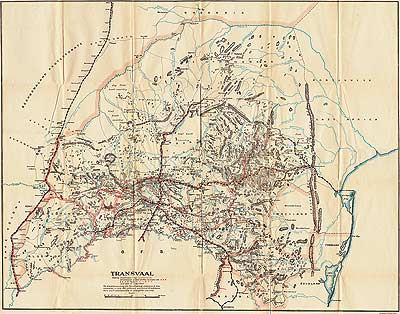This image showcases a vintage, landscape-oriented map of the Transvaal region, characterized by its aged, cream-colored paper showing signs of wear with visible wrinkles and fold lines from top to bottom. The map, likely scanned from an old publication, displays a multitude of black lines representing various routes and features across the terrain, interspersed with highlights in gold, blue, and dark pink. These colored lines intertwine like veins across the map. In the bottom left corner, the map prominently features the text "Transvaal," spelled T-R-A-N-S-V-A-A-L, with an adjacent, smaller paragraph of text and a scale for interpreting the map’s details. The overall style is reminiscent of vintage print cartography, capturing the intricate allure of historical mapping.